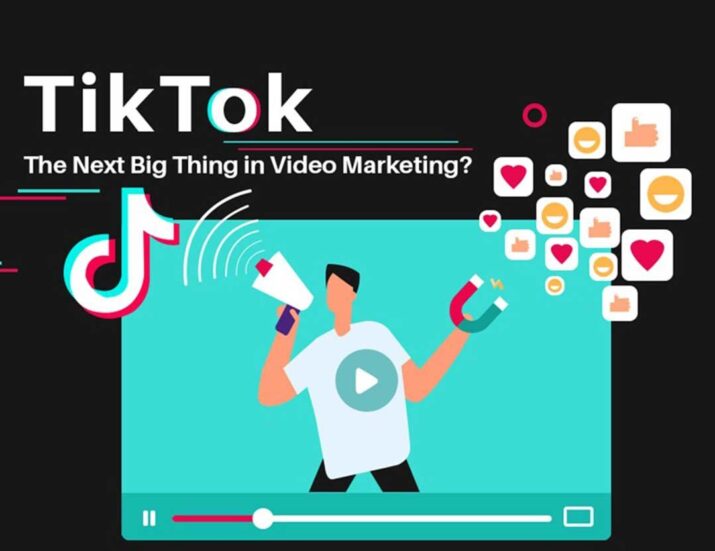"This image appears to be a screenshot from a marketing video themed around TikTok. The background is completely black, providing a stark contrast to the vibrant elements typical of TikTok's branding. Centered at the top, the text reads 'TikTok: The Next Big Thing in Video Marketing,' in white, with a distinctive green and pinkish outline matching the TikTok logo's colors. Below the text, a TikTok symbol is embedded within a green rectangle, which also features a character holding a megaphone with sound lines emanating from it. In the character's other hand is a magnet, symbolizing attraction or drawing in an audience. The character's shirt has a video play button on it, suggesting interactivity.

At the bottom of the image is a progress bar indicating that the video is about one-quarter played. On the right-hand side of the image, there are approximately 15 small boxes with varying icons: about five have thumbs-up symbols, five have hearts, and the remaining five have smiley faces, all in different sizes, adding an element of charm and engagement. This visually appealing and informative snapshot encapsulates the essence of TikTok's influence and potential in the realm of video marketing."